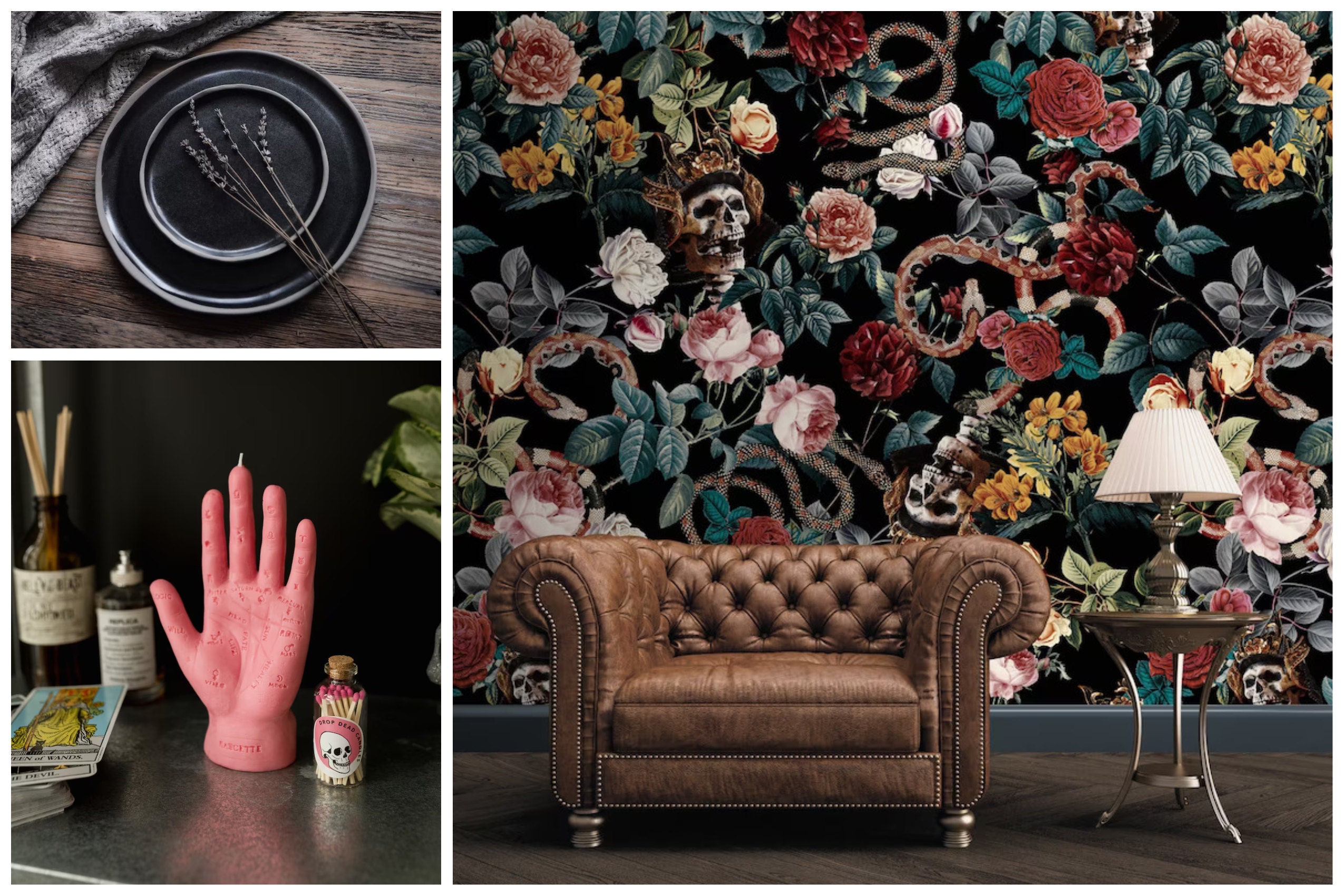This composite image is divided into three sections, each showcasing distinct elements. The left-hand side features two smaller images. In the top left corner, there is a detailed close-up of two black plates—one smaller plate nested within a larger dinner plate—adorned with sprigs of lavender, all set on a dark wooden surface. Above this, a piece of fabric peeks in from the corner. Below this, another square captures a pink, wax hand-shaped candle with a wick on the middle finger, situated on a metal table. Accompanying the hand candle are two brown bottles, a small pile of tarot cards, and a glass jar filled with matches bearing a skull sticker.

The right side of the image, taking up more than half of the entire composition, displays a more elaborate scene. A luxurious brown leather sofa sits on a wooden floor, set against a gothic-inspired wallpaper that features an intricate pattern of roses, skulls, and snakes. To the right of the sofa, a metal stand holds a lamp, adding a vintage aura to the setting. The vivid details and thematic elements of each section combine to create a visually captivating and atmospheric collage.